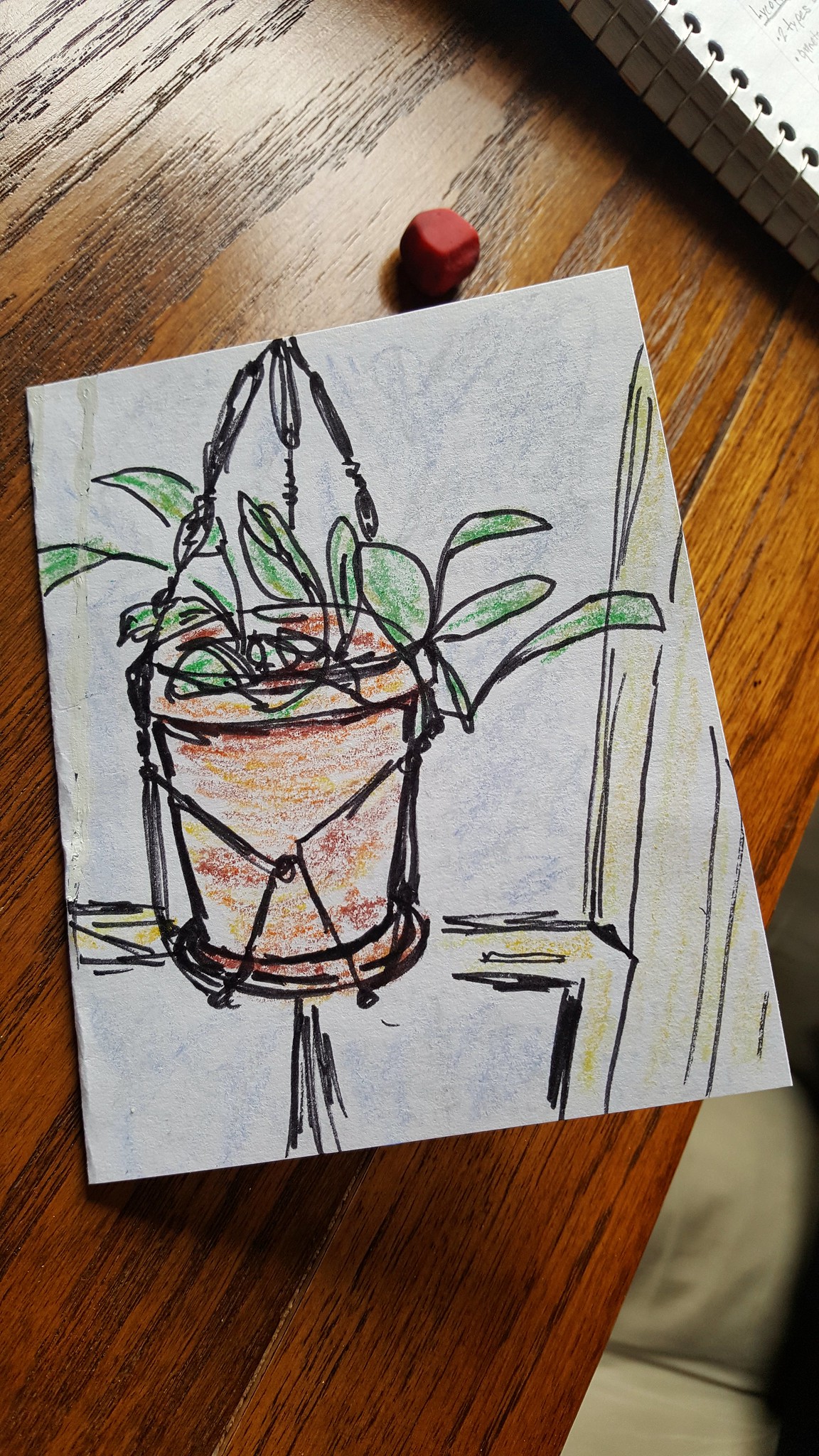The drawing on the white sheet of paper depicts a vibrant green-leafed plant nestled in a red clay pot. The pot is intricately secured with a black rope and suspended using three black chains that converge at a single point, suggesting it's designed to hang. To the right of the plant, a tan-colored structure with vertical black lines stands upright, accompanied by a tan, upside-down, backwards "L" shape. A small, straight tan mark is visible to the left of the pot. Below the plant, five straight black lines descend vertically. Above the paper, a small pink eraser nub protrudes, indicating it's all placed on a brown wooden table adorned with black lines. In the upper right corner, a binder with metal hoops holds the paper together. The bottom right corner reveals some tan cloth with distinctive lines running down the center.